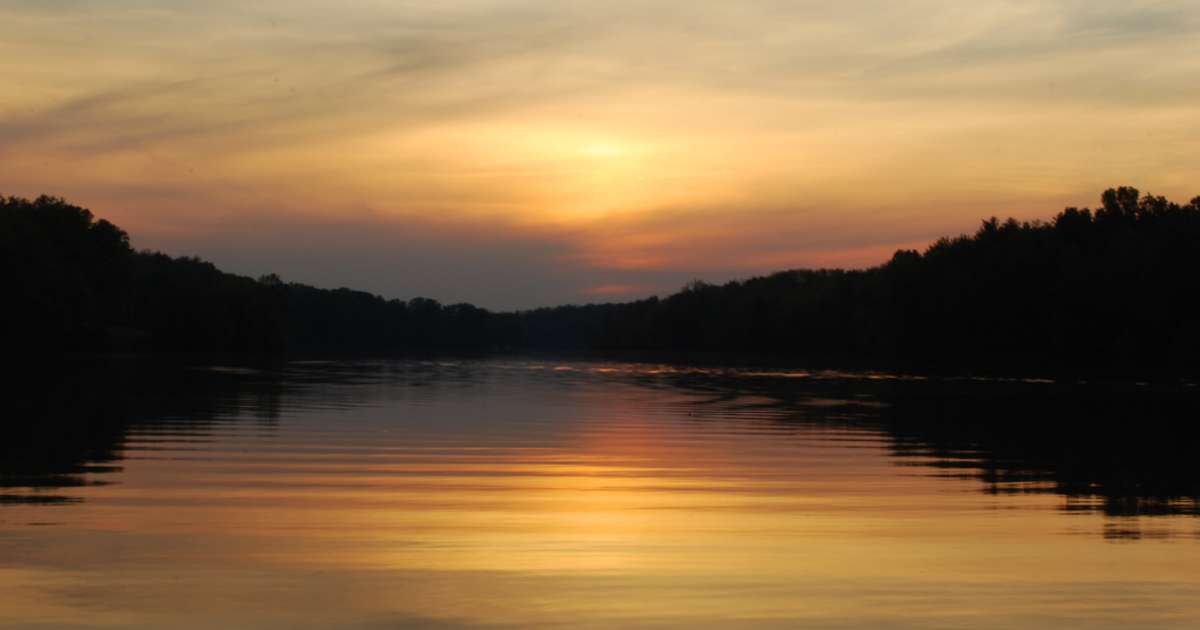This serene landscape photograph captures the evocative beauty of a sunset over a calm lake, enveloped in a spectrum of vibrant hues. The sky is a canvas of striking colors, transitioning from radiant yellows and oranges near the unseen sun to deeper shades of pink, dusty rose, and pockets of light gray and blue where clouds linger. These rich colors are mirrored perfectly in the tranquil waters of the lake, enhancing the moodiness of the scene.

Encircling the lake, a dark fringe of trees stands in silhouette, their black forms outlining the water's edge and adding contrast to the colorful spectacle above. The reflection in the water amplifies the image, with gentle ripples diffusing the brightness of the sunset across the surface and the mirrored contours of the trees creating an almost symmetrical composition. The overall atmosphere is one of quiet solitude and natural beauty, captured just as the last light of day fades behind a curtain of clouds.